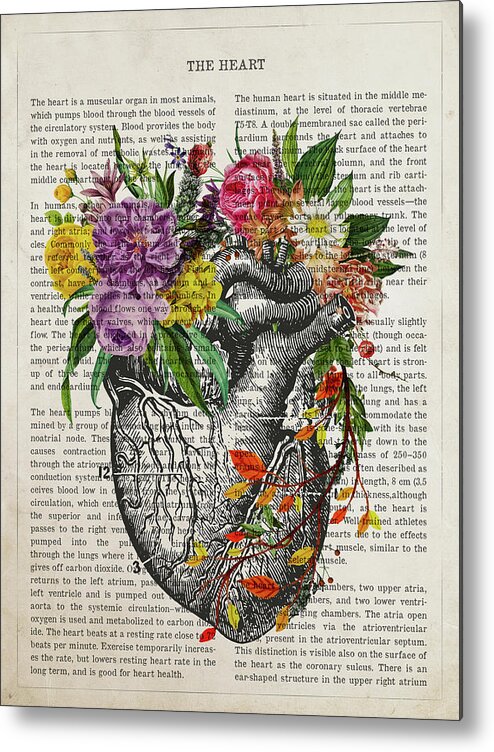The image is a beautifully detailed illustration designed to mimic a page from a book, entitled "The Heart" at the top. The background consists of two columns of typewritten text in an old-fashioned font, providing an in-depth description of the heart as a muscular organ that pumps blood through the circulatory system. This text is predominantly black and white, reminiscent of antique medical illustrations.

Centrally featured on the page is a meticulously hand-drawn, black-and-white anatomical heart, shaded using various pen strokes and lines. The heart serves as a vase holding a vibrant bouquet of wildflowers, offering a stark contrast to the monochromatic background. Among the colorful flowers are a large pink rose, purple flowers resembling daisies or roses, yellow flowers that could be goldenrod, and a white daisy with a yellow center. The greenery includes leaves in various stages of autumn, adding red, orange, and green hues to the composition. Tiny vines with colored leaves extend down the sides of the heart, enhancing the intricate design. This piece artfully combines scientific detail with creative expression, making it suitable for display as framed art.